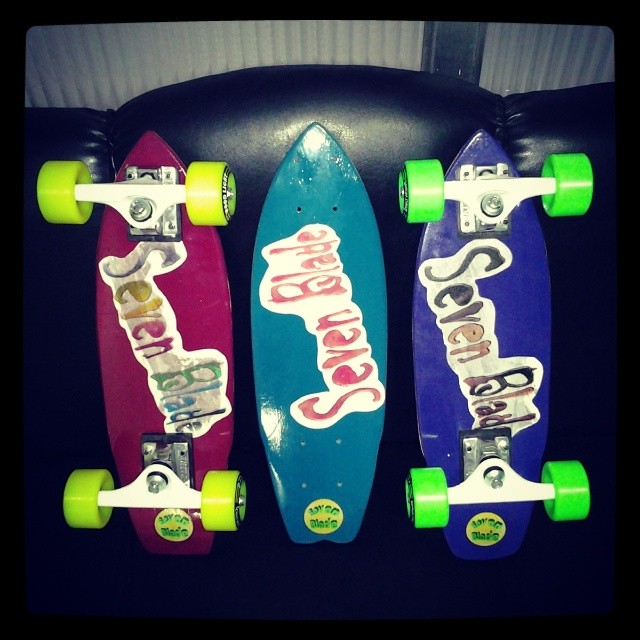This photograph captures three short skateboards leaning against the backrest of a black leather couch. The couch is positioned against a white wall, divided by a small gray slat divider. Each skateboard prominently displays a decal that reads "Seven Blade." The skateboard on the left is a vivid fuchsia pink with neon yellow wheels and features a multi-colored "Seven Blade" sticker. The center skateboard, which lacks wheels, is a bright aqua blue and also bears the "Seven Blade" sticker, seemingly in red ink. The skateboard on the right is a deep royal blue with neon green wheels and, like the others, has a "Seven Blade" decal on its underside.